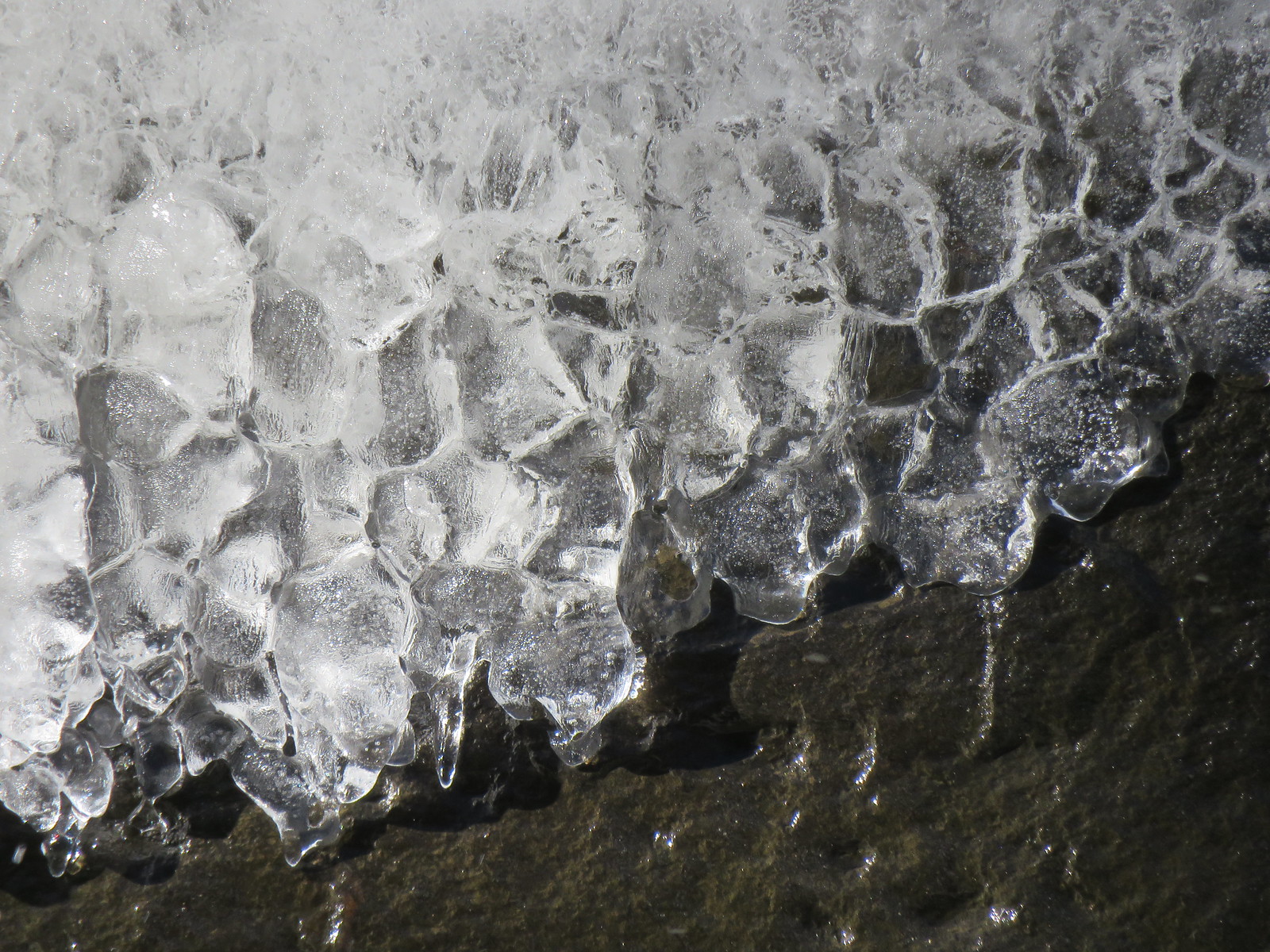This detailed color photograph captures a close-up view of a natural scene dominated by ice and rock. At the center of the image, glistening ice cubes are fused together, some appearing like shards, partially melted under the Sun. This icy formation, slightly dripping water, is set against a rugged, dark grey and brown rock surface, which might have accumulated some dirt. The rock's rough texture occupies the bottom right corner, while the melting ice prominently takes up most of the frame, especially towards the top left. The image is taken outdoors in daylight, likely during winter, showcasing various shades of gray, white, and black, giving it a striking, natural monochrome palette.